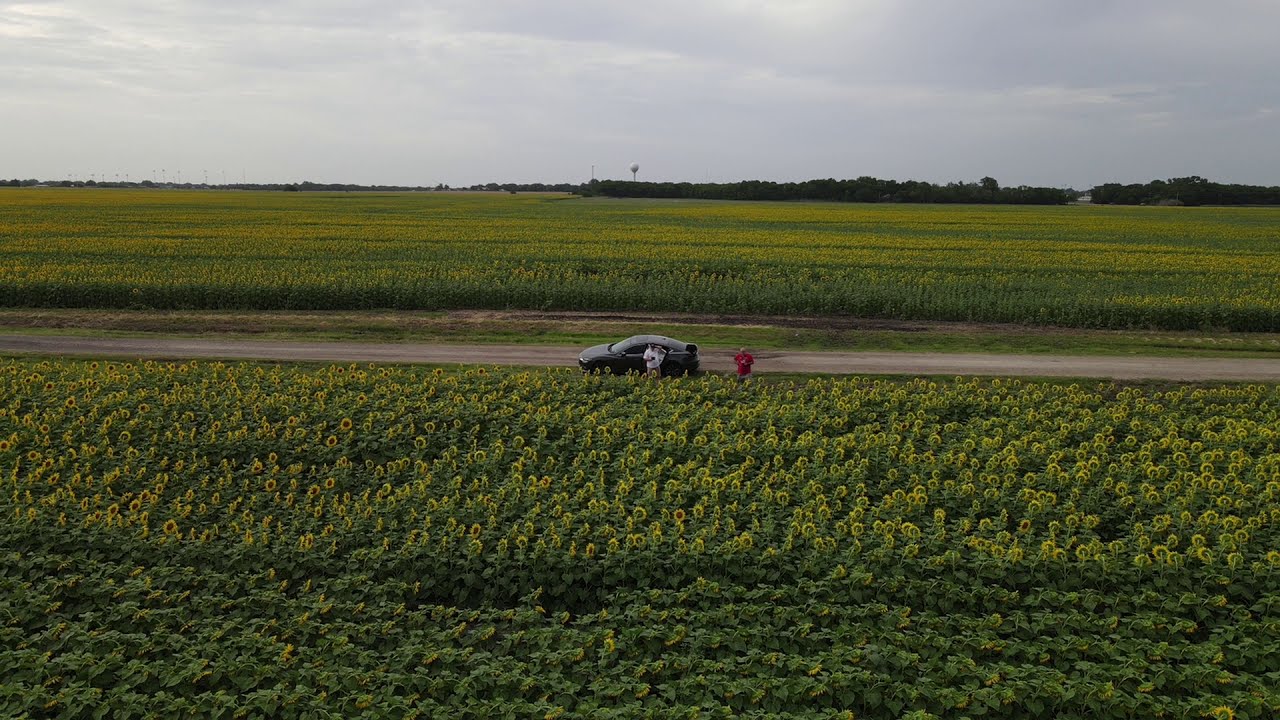The image appears to have been captured from a high vantage point, possibly by a drone, showcasing a large sunflower farm. A road cuts horizontally through the center of the field from right to left. A black car is parked on the side of the road, and two people, one wearing a yellow shirt and the other a white shirt, stand nearby. They seem to be admiring the sunflowers or taking photographs. The vibrant yellow of the sunflowers contrasts beautifully with the green of the field, creating a picturesque scene. In the distance, there is a water tower and some trees, adding to the rural charm of the setting. The sunflowers are densely packed in straight rows, filling the entire landscape with their cheerful blooms.